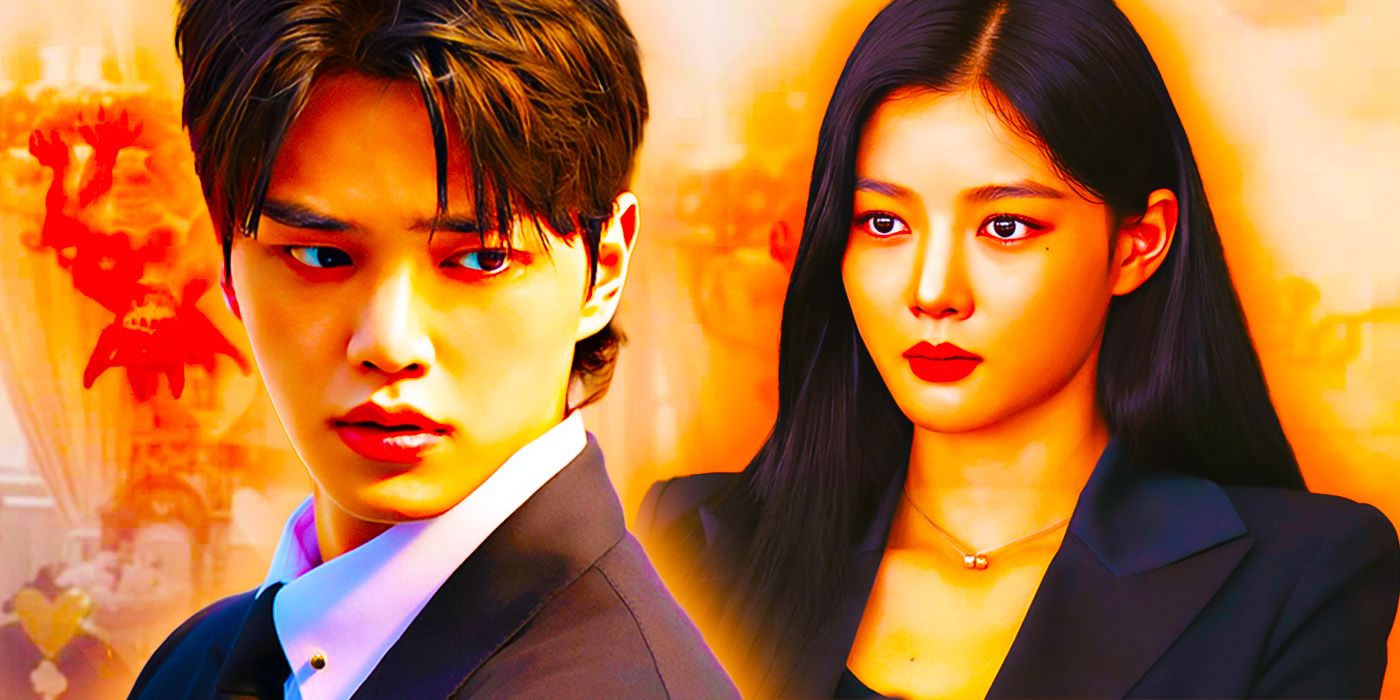The image portrays a cartoon-style depiction of an Asian man and woman against a blurred, orangey-red background with hints of yellow and white. The man, positioned on the left, has medium-length, dark brown hair parted in the middle, slightly brushing over his eyes, and is sporting flat black eyebrows and large lips. He appears upset or worried, looking over his shoulder towards the right, with dark brown eyes fixed on the woman. He is dressed in a white button-down shirt with a tie, beneath a black dress coat.

On the right, the Asian woman has long, straight black hair parted in the middle, showcasing thin eyebrows and dark eyes. She is adorned with red lipstick and wears a low-cut top under a black blazer. Around her neck is a delicate gold necklace featuring two heart shapes. She seems to be gazing back at the man. Both figures are illuminated by a subtle glow, suggesting that they might be characters in a promotional image for a show, potentially involved in a dramatic moment of their relationship. In the background, abstract red and yellow patterns enhance the emotive and vibrant tone of the scene.